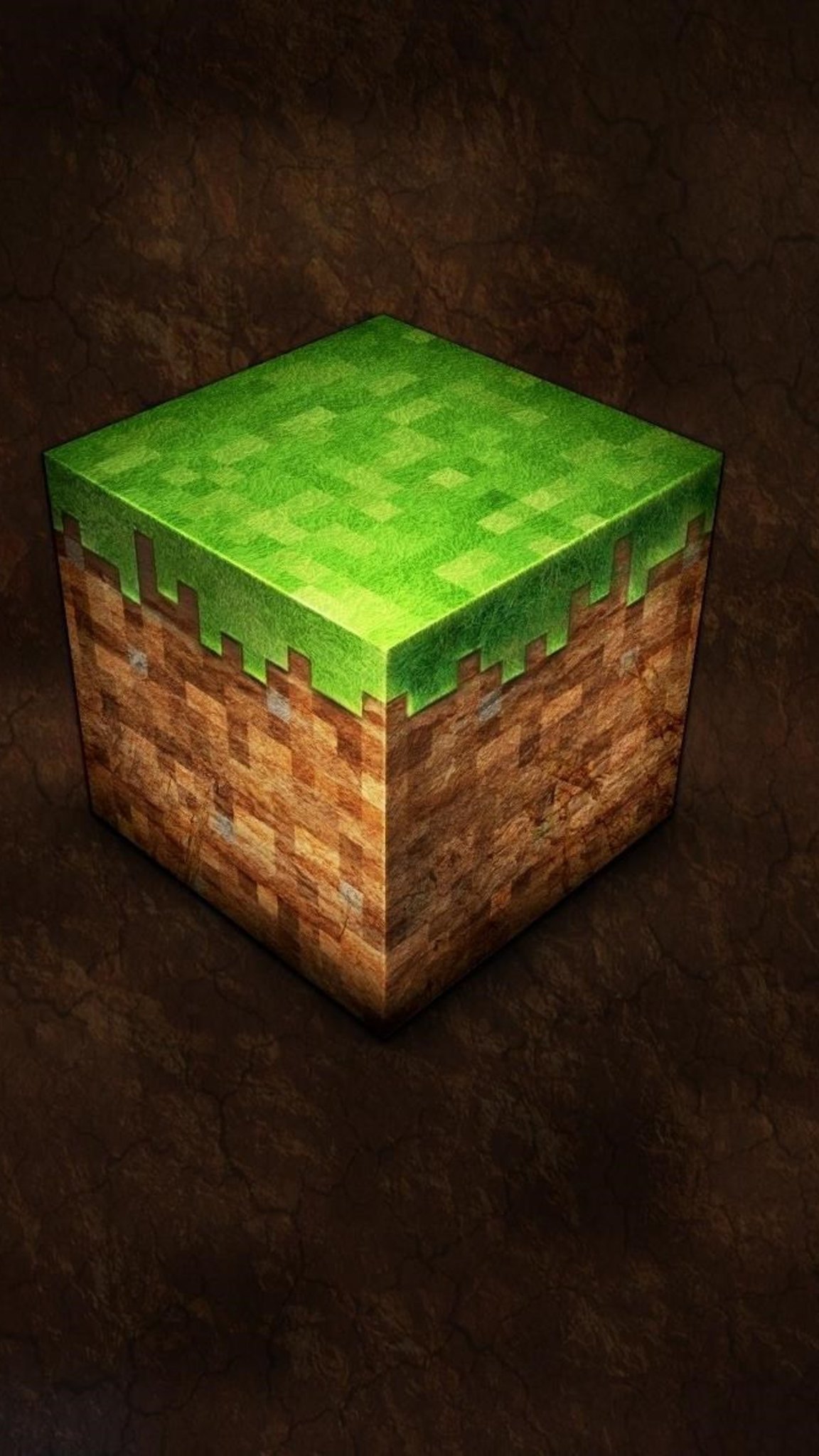This image appears to be a computer-generated representation of a cubic puzzle set against a black background. The cube is divided into two distinct sections: an upper and a lower part. The upper section is a square in vibrant hues of lime green with some darker green accents. It possesses intricately designed grooves on all sides, which align perfectly with the lower section, indicating it fits snugly like a puzzle piece. The lower section of the cube displays various shades of brown, ranging from tan to deep brown, giving a textured appearance. The overall visual effect creates an impression of a meticulously crafted 3D puzzle where the top green piece must fit precisely into the brown base. The stark black background highlights the contrast between the bright greens and earthy browns, emphasizing the cube's detailed design and puzzle-like nature.